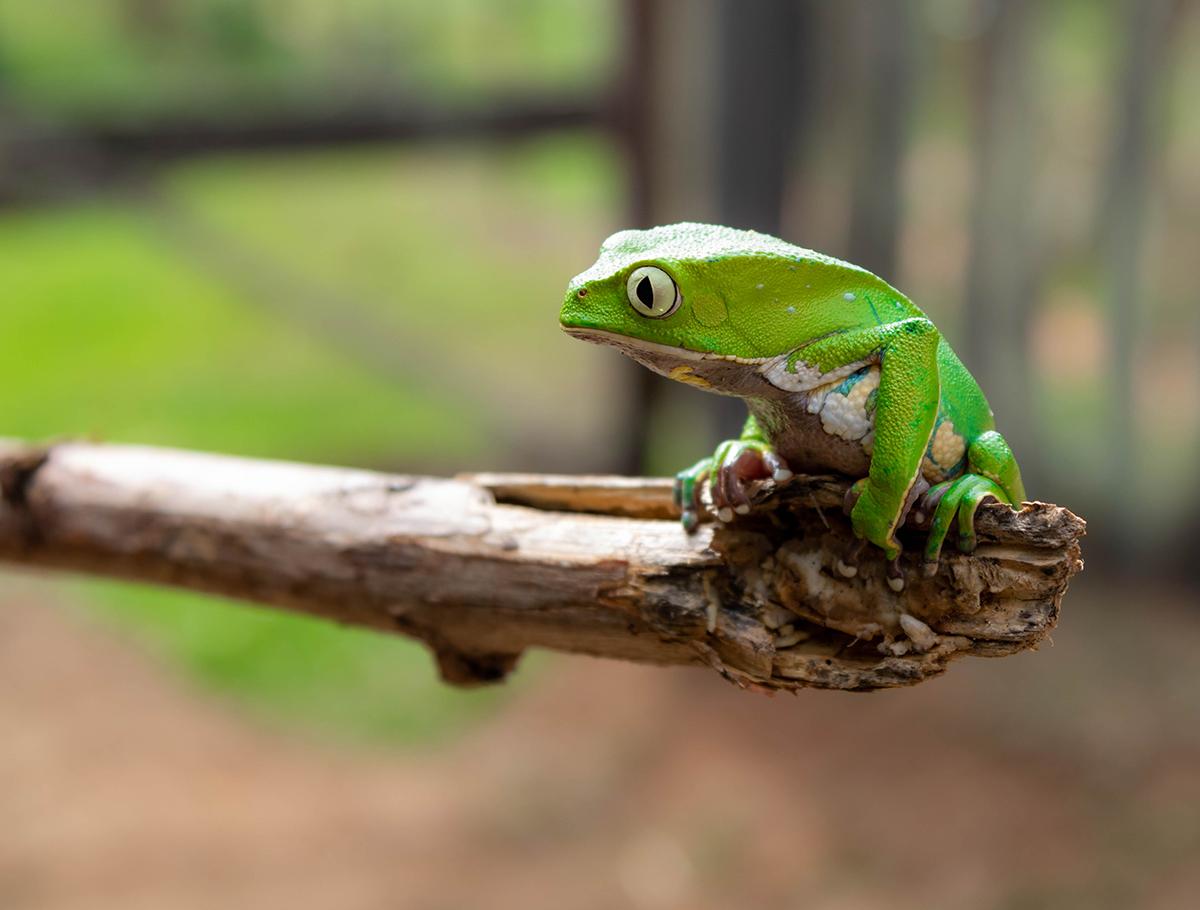The photograph captures a vivid lime green frog perched at the very edge of a brown wooden branch. The frog is facing towards the left, displaying a side view of its left profile with an intricate focus on its features. Its eyes are a pale green with prominent black slits for pupils, and it seems as though the frog is aware of the camera, perhaps even looking directly at it. The tips of its fingers and toes are distinctively white, resembling painted fingernails. The underbelly of the frog shows a mix of dirty brown streaks, suggesting it has recently been in mud, along with patches of lighter orange, yellow, and blue hues. The background of the image is blurred, highlighting the frog and the branch while hinting at an out-of-focus scene that includes some patches of grass, a fence, or possibly a gate in the distance. The frog's vibrant green color contrasts sharply with the muted background, making it the focal point of the photograph.